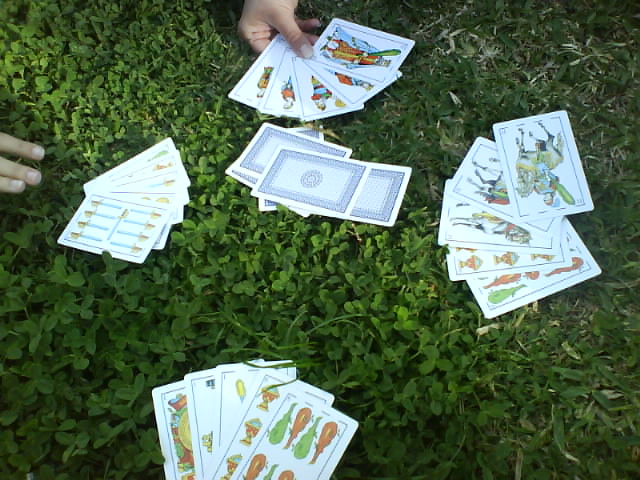In this vibrant photograph, we observe a card game in progress on a lush green grass backdrop. The grass spans the entire background, exhibiting some whitish patches particularly noticeable in the top right corner. In the top section of the image, a hand is gripping five cards, positioned in a way that suggests engagement in an ongoing game. Three fingers appear on the left side, aiding in presenting six cards laid out on the grass nearby. Toward the right, another set of five cards rests on the grass, while at the bottom, four more cards are arranged. These scattered cards display an array of images; notably, the top right card depicts a person riding a horse, giving a glimpse into the possible thematic elements of the game. On the left, the uppermost cards showcase symbols, such as a card adorned with nine swords. Centrally located is a deck of cards, facing down, adding to the sense of anticipation in the game. The detailed imagery on the cards, including people and various symbols, hints at a possibly intricate and engaging card game being played in this serene outdoor setting.